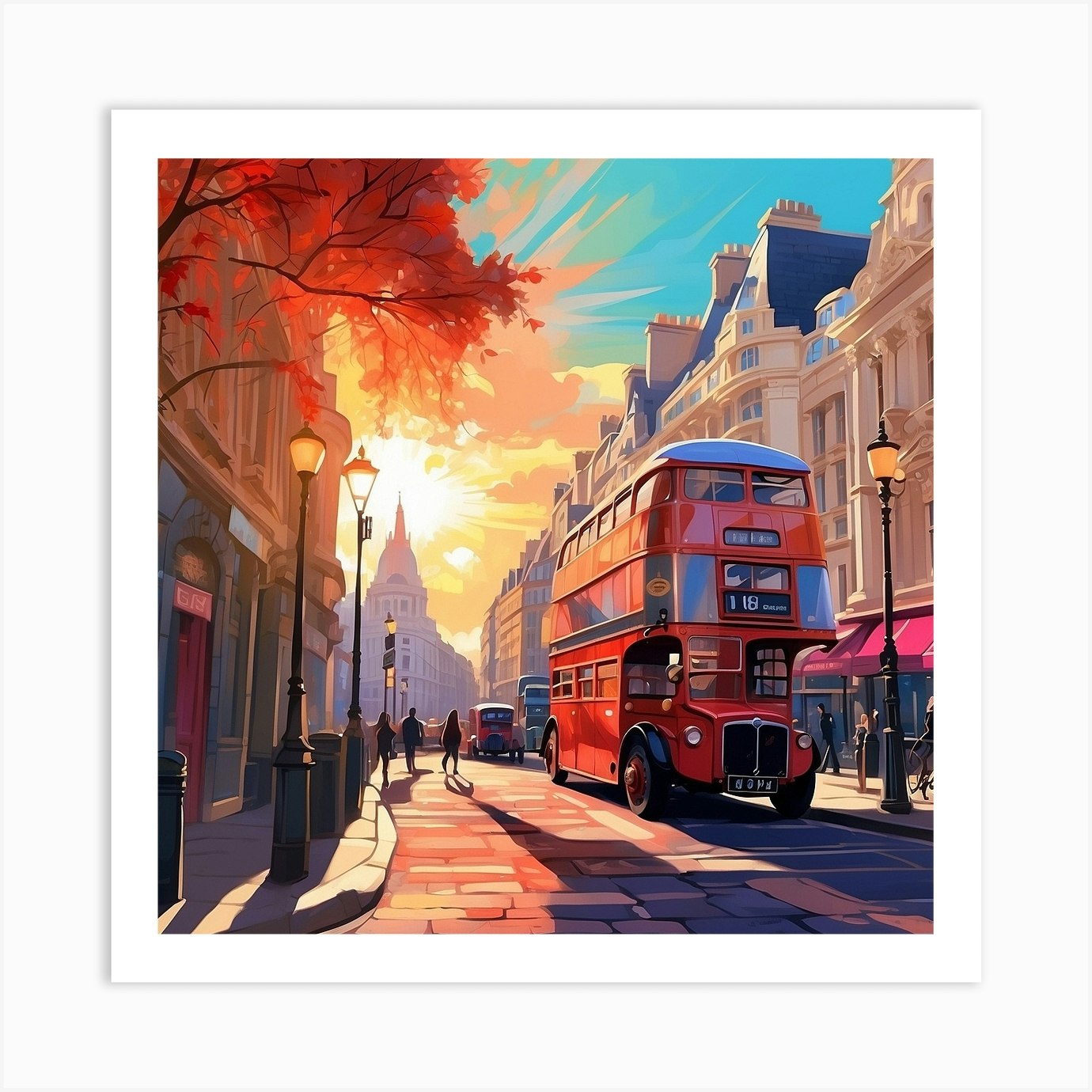This image resembles an impressionistic travel poster depicting a lively city scene bathed in bright sunlight. The sky is a vibrant canvas of blue, interspersed with shades of white and yellow, with a radiant yellow sun casting shadows across the landscape. Dominating the scene is a red double-decker bus, which is captured as it moves towards the viewer along a cobblestone street, accompanied by a lorry trailing behind it. Pedestrians dot the scene, with three figures walking on the left side and another person visible on the right, possibly near a parked bicycle.

In the top corner, an orange, autumnal tree adds a splash of color. The setting is framed by buildings on either side of the street, some adorned with red awnings. Street lamps, both lit and casting shadows, further emphasize the sunny day. The buildings, appearing to be two-story apartments and commercial establishments, add depth to the bustling atmosphere of this cityscape. This richly detailed image, whether painted, drawn, or computer-generated, captures the essence of a sunlit day in a vibrant city square.